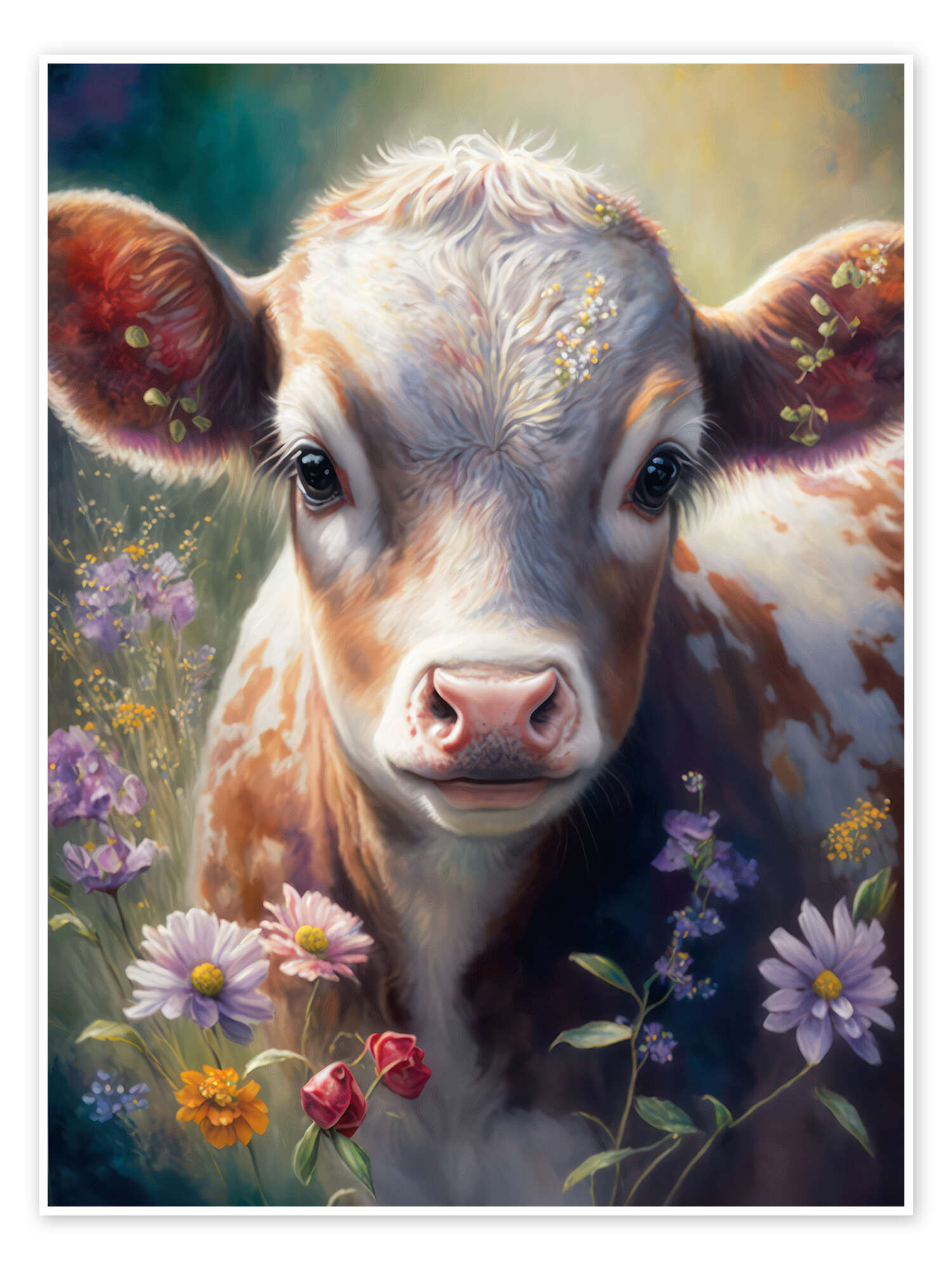This image is a serene and peaceful painting of a young calf, prominently centered in the frame. Painted in HD with soft, muted colors and a gentle glow, it exudes a springtime fantasy feel. The calf, with a predominantly white face and a pink snout, showcases brown spots across its body and a tuft of white fur on its head. Its large, dark eyes brim with reflected light, framed by light, prominent eyelashes, giving it an endearing and cute appearance. The ears extend towards the edges of the image, with some flowers resting on them, contributing to the whimsical charm. The background hints at a meadow with a variety of vibrant wildflowers in bloom, featuring purple, yellow, pink, orange, and red flowers. The hazy, pastel style and the detailed depiction of the flora and fauna create a dreamy and serene composition, making the calf appear as though it is part of a fairytale landscape.